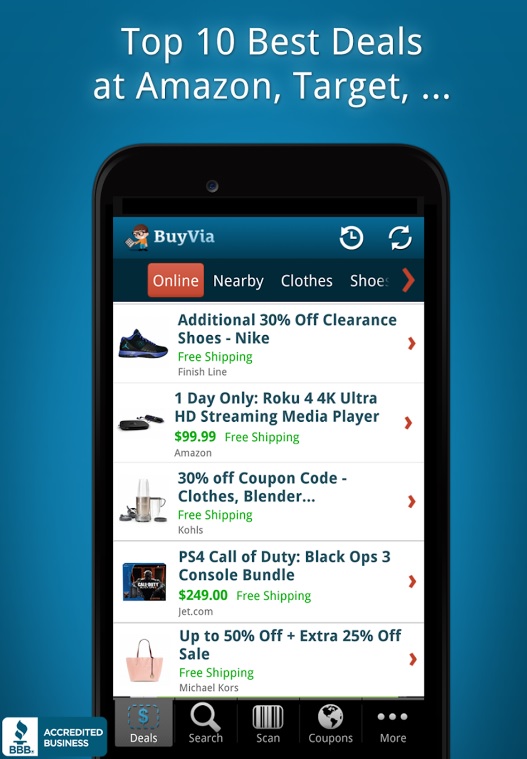The image features a blue vertical rectangular screen as the background. At the top, on the blue background, is a white text reading "Top 10 Best Deals at Amazon, Target, and ..." Below this, centered on the screen, is a picture of a cell phone. The phone's model is black and it displays a website named "Buy Via" at the top.

Just below the website name is a navigation menu with options labeled "Online," "Nearby," "Clothes," and "Shoes." The "Online" tab is highlighted with a red rectangular box. This menu is followed by a list of items for sale, each title in blue text. Below each title, the shipping cost or free shipping details are indicated in green, with the store name in small gray font underneath.

The list of items starts with a picture of a shoe, accompanied by the text "Additional 30% Off Clearance Shoes Nike Free Shipping Finish Line," indicating the store, not the brand. Below the shoe image is a picture of a Roku device, with the description "One Day Only Roku 4 4K Ultra HD Streaming Media Player $99.99 Free Shipping Amazon." Next is an image of a blender, detailed with "30% Off Coupon Code Clothes Blender Free Shipping Kohl's." Following the blender, there's a picture of a PS4 gaming console with "PS4 Call of Duty Black Ops 3 Console Bundle $249 Free Shipping Jet.com." The final item presented is a bag, labeled "Up to 50% Off Plus Extra $25 Off Sale Free Shipping Michael Kors."

At the very bottom of the cell phone screen are five buttons arranged from left to right labeled "Deals," "Search," "Scan," "Coupons," and "More." Additionally, on the bottom left corner of the blue section of the overall image, there's a small white and blue rectangle displaying "BBB" and underneath it "Accredited Business."